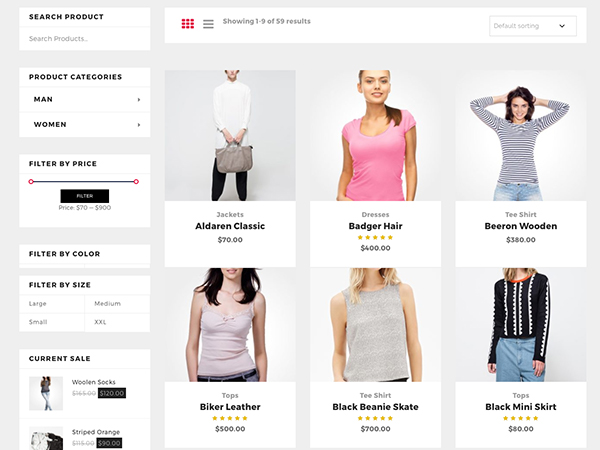In this image, we are viewing a clothing website interface with multiple product listings. The top of the page displays navigation information indicating "Showing 1 of 9 of 59 results," yet only six images of women modeling various outfits are visible.

1. **Top Row (Left to Right):**
    - A woman wearing a white jacket, priced at $70.
    - Another image features a woman in what appears to be a pink dress, priced at $400, although initially referred to as a shirt.
    - To the right, a woman is seen in a striped maroon t-shirt listed at $380.

2. **Bottom Row (Left to Right):**
    - There is a listing described as a black miniskirt, but the image shows a woman in Levi's jeans priced at $80.
    - Next, a product labeled "black beanie t-shirt" is shown, but the actual picture displays a woman in a gray tank top.
    - Lastly, another listing titled "biker leather" features yet another gray tank top worn by a different woman.

Additional features of the website include filters by color, gender (man and woman), and size. However, the brand or store name is not visible within the image.